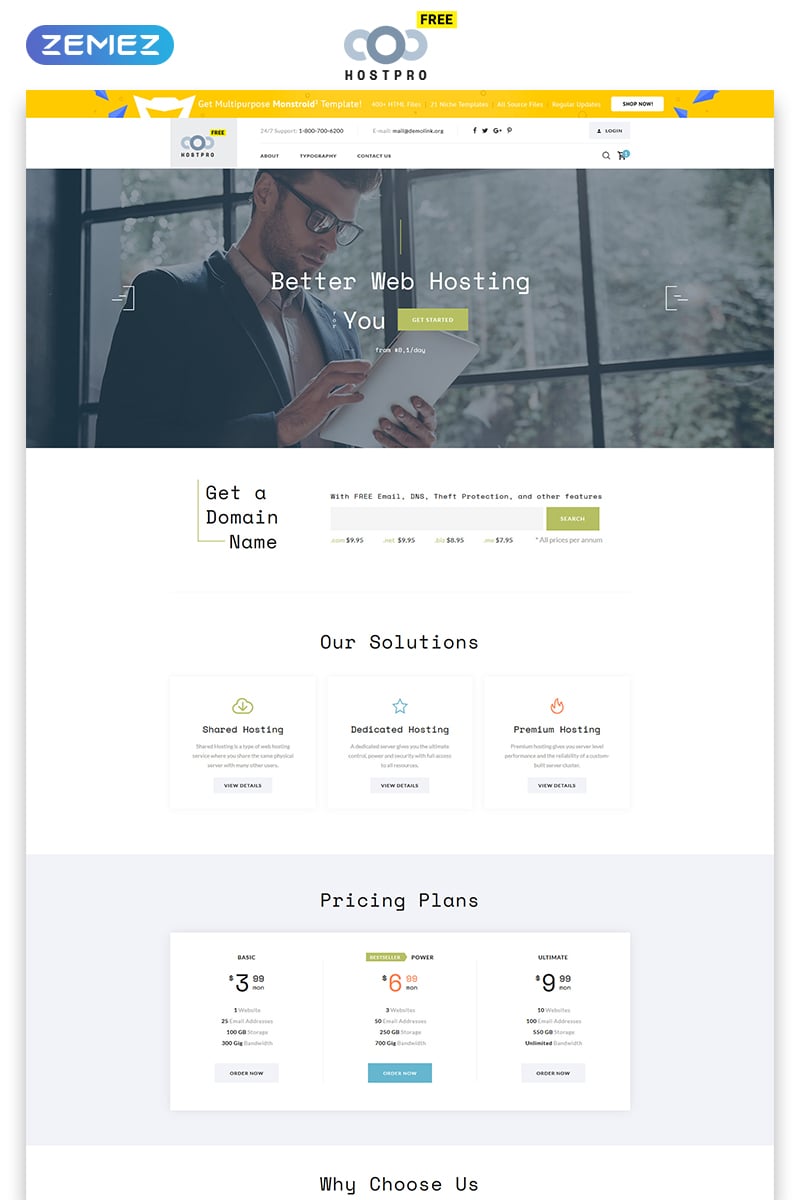This image features a web page for a hosting service called "Zemez," prominently displayed at the top left corner within an elongated blue circle with white lettering. In the middle at the top, it says "Host Pro" in black text beneath a series of interlocked curvy lines with a central circle, all in varying shades of gray. To the upper right, there's a yellow box with the word "FREE" in black text.

At the top of the page, there is a call-to-action box for searching domain names, emphasizing the website's focus on web hosting services. A central image shows a young man in his 20s, dressed in a business jacket over a shirt with no tie and wearing dark glasses. He is holding a tablet in his left hand and interacting with it using his right hand, standing in front of windows that reveal a backdrop of trees outside.

Midway down the page, a section titled "Our Solutions" features three distinct boxes. The first box, labeled "Shared Hosting," includes a brief description and a "View Details" button. The middle box is for "Dedicated Hosting," also with a "View Details" button. The third box on the right is for "Premium Hosting," and similarly includes the "View Details" button.

Below this section is a pricing table displaying different plans. The "Basic" plan is priced at $3.89 per month and lists included features. The "Power Option" plan is priced at $6.99 per month and is marked with a flag indicating it is a best-seller, along with its respective features. The "Ultimate" plan is at $9.99 per month, detailing its additional features.

At the bottom, although the text is cut off, the bold black words "Why Choose Us?" are visible, indicating a section likely dedicated to explaining the unique selling points of the service. The image ends mid-content, leaving some elements incomplete.